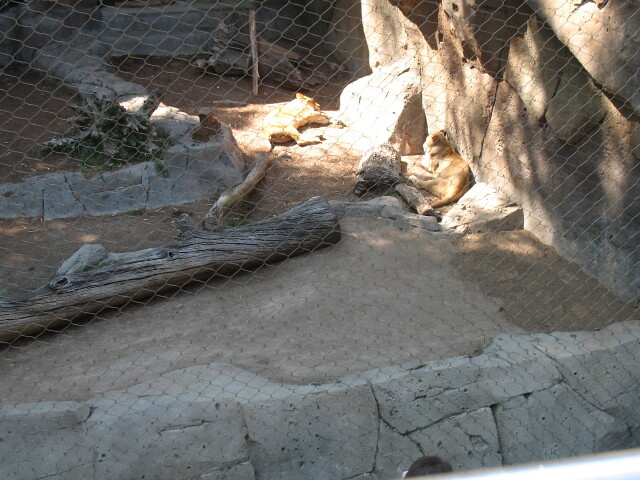The photograph captures a zoo enclosure encircled by a tall chain-link fence, which includes stones, a fallen log, and a concrete wall. Two light-colored female lions (or large cats) are seen lounging in the enclosure. One lion is stretched out on her left side, basking in a sunlit patch of ground, while the other is reclining with its head raised against a high outcrop of large rocks, nearly blending into the background. The setting includes additional concrete structures and dirt, creating a naturalistic habitat for these big cats. The image, taken from a distance, also captures the top of a visitor's head at the bottom, peering through the fence into the enclosure.